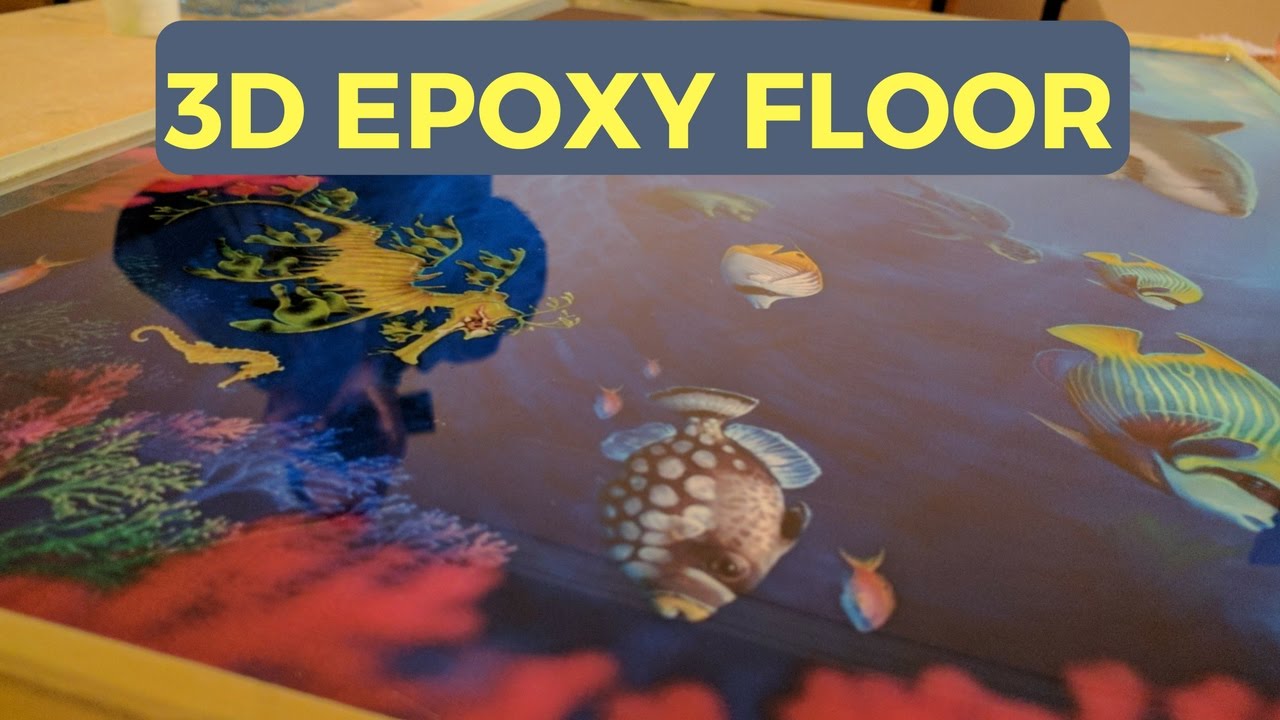This highly detailed advertisement showcases an underwater-themed 3D epoxy floor. The central focal point of the image features a realistic drawing of an ocean scene, complete with various sea creatures and vibrant coral. Among the vividly colored coral—red, green, blue, and pink—there's a distinctive bluish fish with a yellow tail on the right side. Staring directly at the viewer from the center is another blue fish with a speckled underside, adorned with brown and gray spots. Dominating the top of the image, in bold pale yellow text on a contrasting blue background, is the title "3D Epoxy Floor." Just beneath the text is a prominent yellow seahorse with intricate, spindly parts that gradually fade to green. Nearby, a much smaller seahorse is also visible. Additional marine life includes a distant shark, a turtle, a brown fish with white spots, several small pink fish, and a blue and yellow striped fish, all contributing to the vivid, immersive underwater tableau.